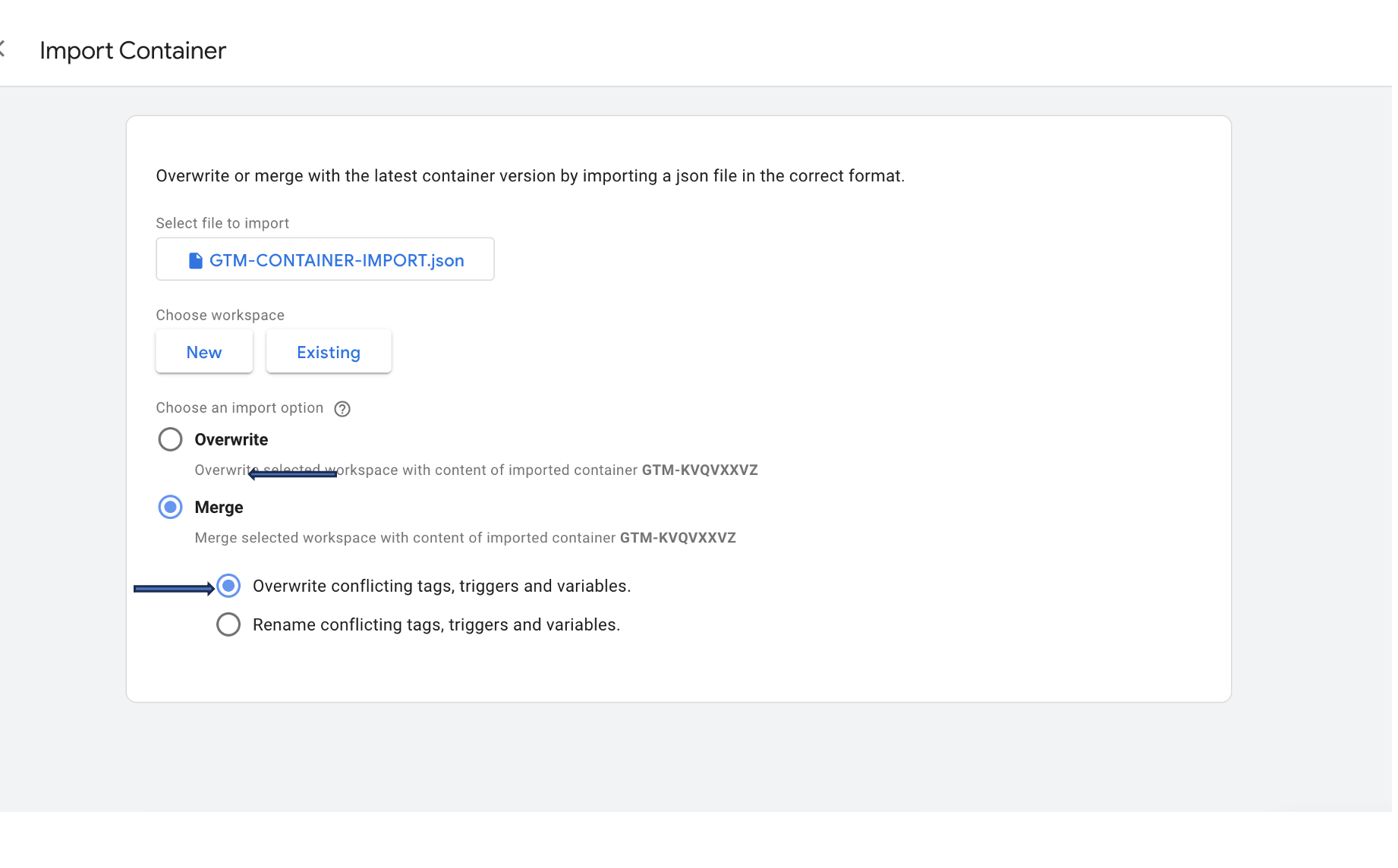The screenshot displays the settings screen of an "Import Container" feature, set against a white background with several lines of text clearly visible. At the top, the title "Import Container" is prominently displayed, accompanied by a faint icon or possibly parentheses on its left side. There are no window taskbar or navigation bar elements visible, making it difficult to determine the exact website or application.

The instructions below the title read: "Overwrite or merge with the latest container version by importing a JSON file in the correct format." Underneath, there's a prompt to "Select file to import," showcasing a selected file labeled "gtm-container-import.json."

Following this, users are prompted to "Choose workspace," with the options being "New" or "Existing." Below this section, there's a directive to "Choose import option," offering two choices. The first option is "Overwrite/New Workspace with content of imported container," which has been partially struck through, hindering full readability. The second option is "Merge," defined as "Merge selected workspace with content of selected container."

Towards the bottom of the screen, an arrow highlights the selected preference, "Overwrite conflicting tags, triggers, and variables." Additionally, an unselected option reads, "Rename conflicting tags, triggers, and variables." This comprehensive overview provides a lucid depiction of the import process for container settings.